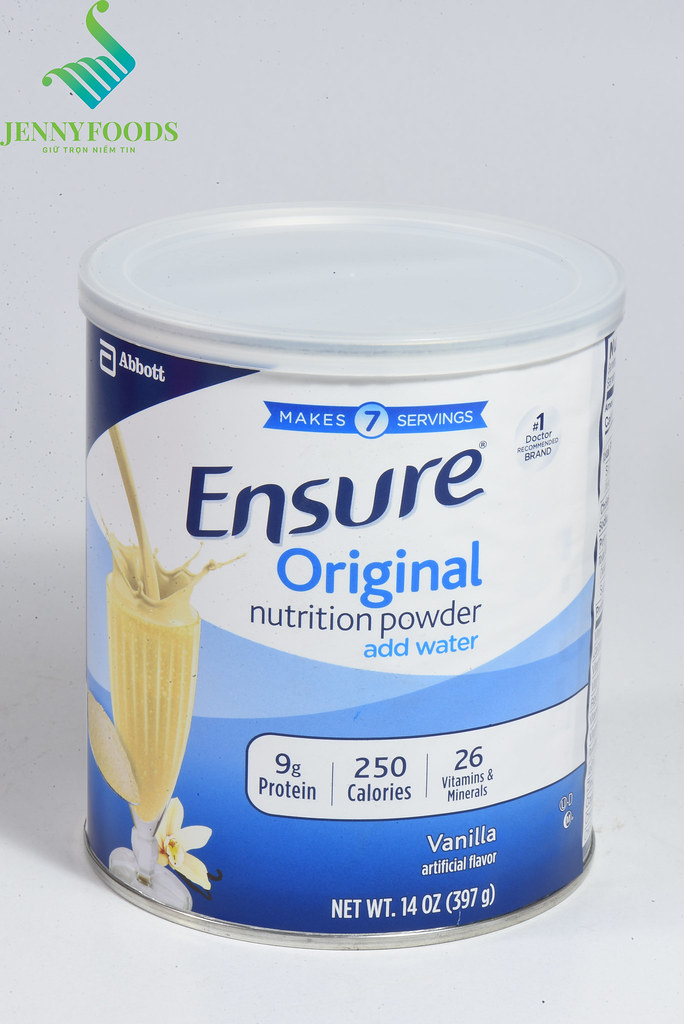In the image, a cylindrical canister is placed on a white surface with a white background, creating a clean and minimalistic setting. The top left corner of the image features a logo labeled "Jennifold" in green text, with "Gimtron Niemtin" written below it, also in green. The logo incorporates shades of green along with hints of blue.

The canister itself is adorned with a white sticker that displays an intricate design featuring various shades of blue, ranging from light blue to dark blue. The canister is sealed with a plastic lid that is slightly gray in color. The sticker prominently indicates "Makes 7 servings" in blue text.

Centrally positioned on the sticker is the brand name "Ensure" in bold blue letters, with "Original Nutrition Powder" written below it in a mix of dark blue and blue colors. To the top left of the brand name is the phrase "A Pot." Beneath this text, there is a visual depicting a yellow shake being poured into a glass, accompanied by a spoon on the left side and a flower to the right of the glass.

Further down the sticker, nutritional information is listed: "9g protein," "250 calories," and "26 vitamins and minerals," all in blue text. The flavor is described as "Vanilla Artificial Flavor" in blue letters, and the net weight of the product is specified as "14.0 oz" (397 grams).